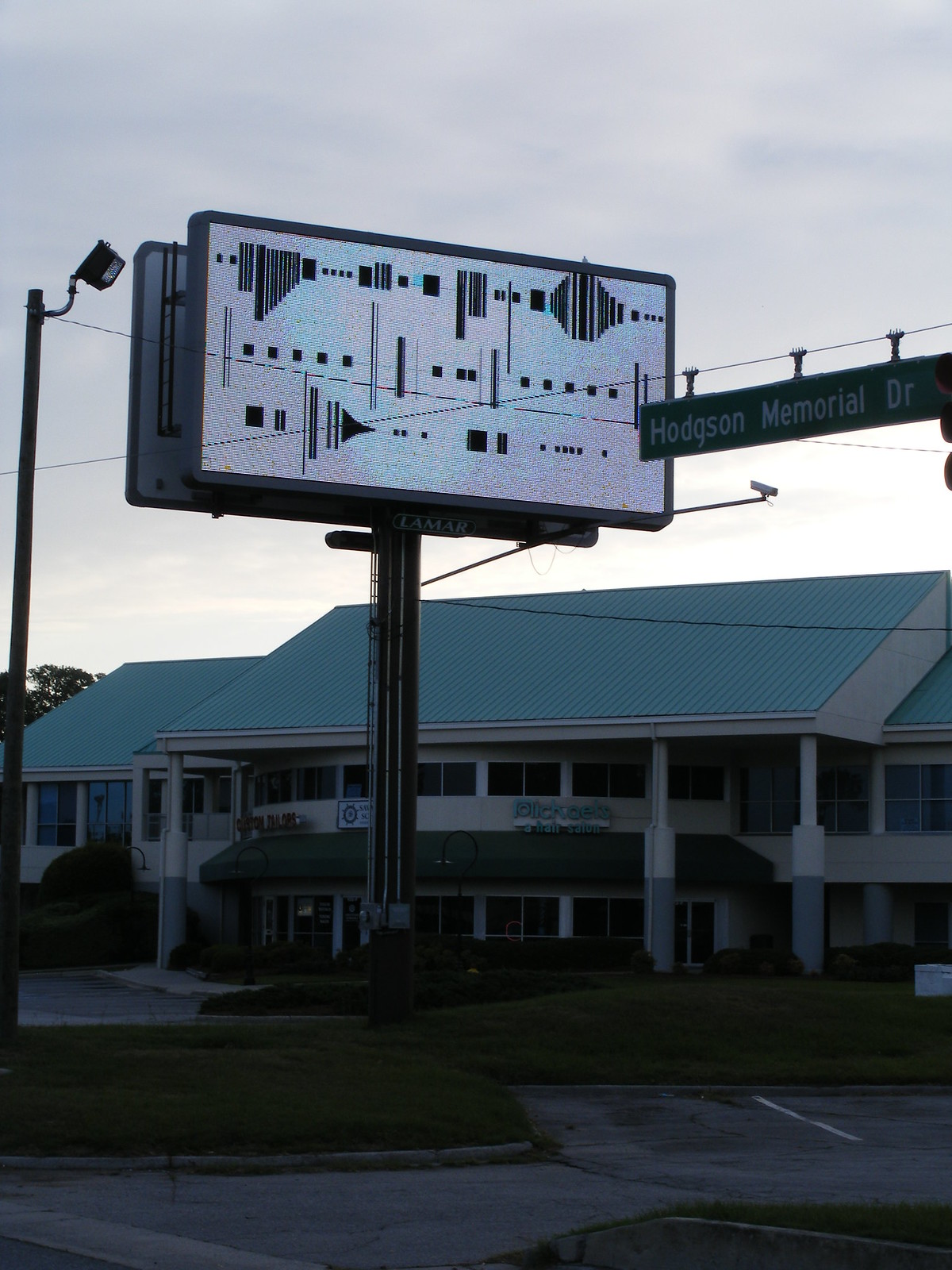This image depicts a tall, vertically oriented photograph taken outdoors on a dimly lit, cloudy day. Dominating the foreground is a large billboard situated approximately 40% in from the left side and starting about 25% up from the bottom. The billboard itself is about halfway up the image and features a white background with an intricate pattern of black lines and shapes resembling sound waves or geometric forms, spanning three rows. 

Directly behind the billboard stands a two-story building, possibly a hotel or convention center, characterized by a teal or brown roof, numerous windows, and a front entrance supported by pillars. Detailed features such as double doors and story-high windows on the first floor can be observed, though they are dimly lit and difficult to discern clearly.

In the background, there's a cloudy sky above a parking lot marked with a white line, alongside grassy areas. To the right of the billboard, a street sign reads "Hodgson Memorial Drive" in white lettering. Additionally, a street light is positioned on the left side of the image.